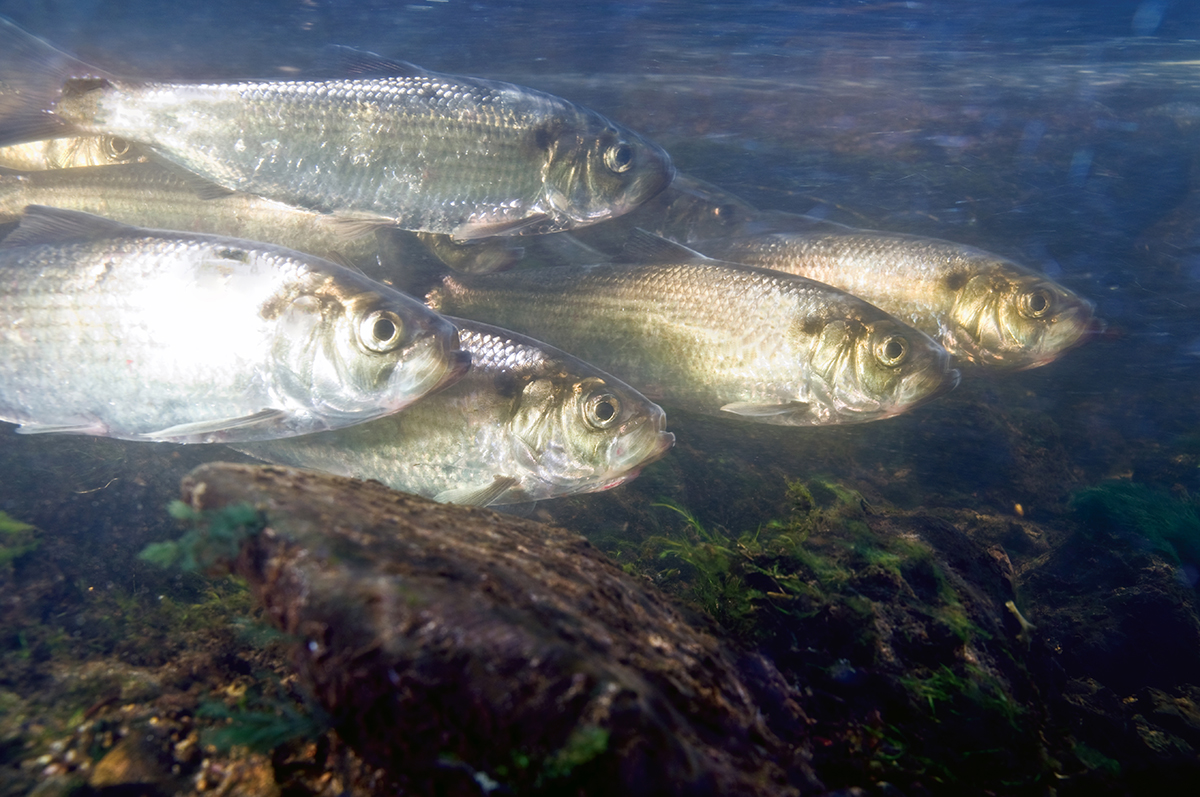This photograph captures an underwater scene featuring a school of small, silverish fish with large black eyes accented with white. They are approximately two inches in length and number between eight and nine, some of which are partly out of the frame. These fish swim close to a rocky bottom covered with green seaweed, algae, and various brown materials, such as mold, dirt, and rocks. The background water has a bluish tint, suggesting the photo is taken either in a natural body of water or a well-maintained fish tank at home. A darker black rock is noticeable on one side, and nearby, there is something resembling either a large log or a lizard-like shape. The surface of the water is indistinct, with light dots visible near the top of the frame. The setting could be an ocean, a river, or a lake, though there's no specific identifying information about the location.